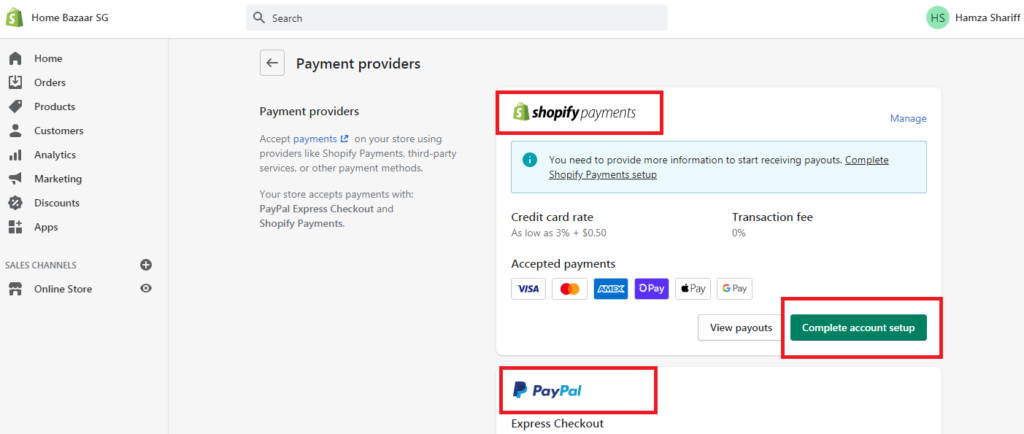Screenshot of the Shopify Dashboard: Detailed View of Payment Providers Section

The screenshot showcases the Shopify Dashboard. In the top left corner, the Shopify logo, represented by a shopping bag with a dollar sign, is visible alongside the store's name, "Home Bazaar SG." At the top center of the screen is a search bar function, facilitating quick access to various features. Towards the top right, the user icon, a green circular element with the initials "HS," indicates the active user, Hamza Sharif.

On the left sidebar, a vertical menu displays an array of navigational tabs: Home, Orders, Products, Customers, Analytics, Marketing, Discounts, Apps, Sales Channels, and Online Store. These tabs provide quick access to different functional areas of the Shopify platform.

Dominating the main section of the screen, spanning from the middle to the right, is the "Payment Providers" module. An informational arrow points to this section. The section starts with a description stating, "Payment Providers accepts payments on your store using providers like Shopify Payments, third-party services, or other payment methods."

The current payment providers for the store are listed as PayPal Express Checkout and Shopify Payments. Notably, Shopify Payments is highlighted by a rectangular box outlined in red, indicating its selection status.

Beneath this, a notification informs the user, "You need to provide more information to start receiving payouts, complete Shopify Payments setup." This directive is underlined and encased within a light blue rectangle, emphasizing the urgency of this task.

Further down, details about credit card transaction rates are provided, stating, "Credit card rate as low as 3% plus 50 cents. Transaction fee is 0%." Directly below, a green "Complete Account Setup" button is enclosed by a red rectangle, prompting the user to finalize the setup process. Additionally, the PayPal name and logo, also highlighted with a red rectangle, denote its inclusion as a payment option, followed by the label "Express Checkout."

The detailed layout and highlighted elements within this screenshot guide the user through the essential steps required to set up and manage payment providers on the Shopify platform.